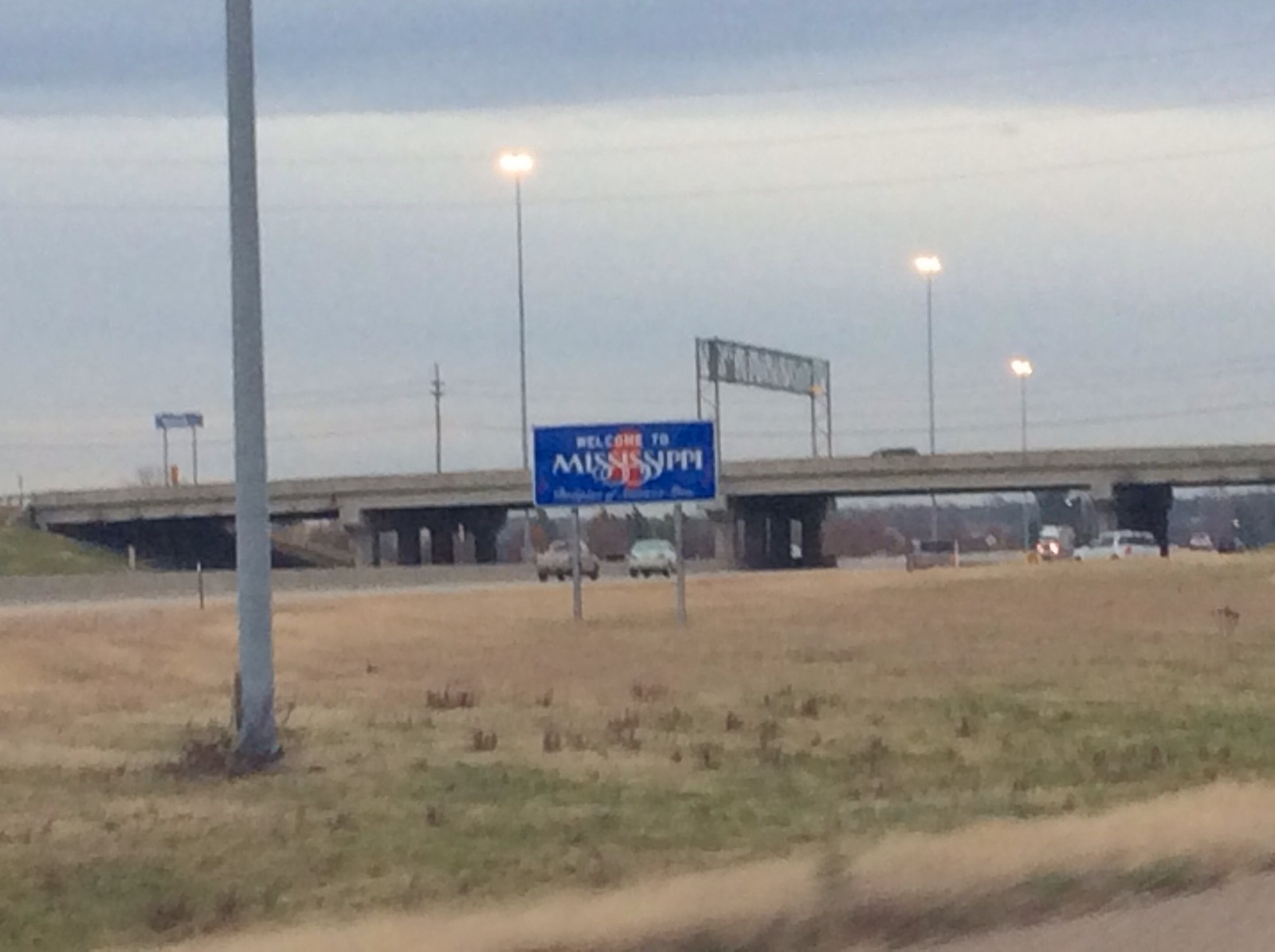The roadside scene captures a bustling highway with various elements. In the foreground, a well-maintained curb borders a sprawling green lawn. Dominating the scene is a prominent light pole, flanked by two smaller poles that support a blue sign with white lettering, welcoming visitors to Mississippi. The sign reads, "Welcome to Mississippi," standing out crisply against its blue backdrop. Further in the distance, a hint of red is visible, though its details are obscured. The highway is alive with traffic, highlighted by a large truck approaching with its headlights shining brightly. A substantial bridge arches over the roadway, accompanied by a series of street lights and power lines strung along a row of poles. The background is rich with tall, leafy trees that add a touch of nature to the otherwise industrial landscape. Adding to the commercial feel of the scene, a large Walmart sign, mounted high on two massive poles, looms on the horizon, its blue background easily identifiable.